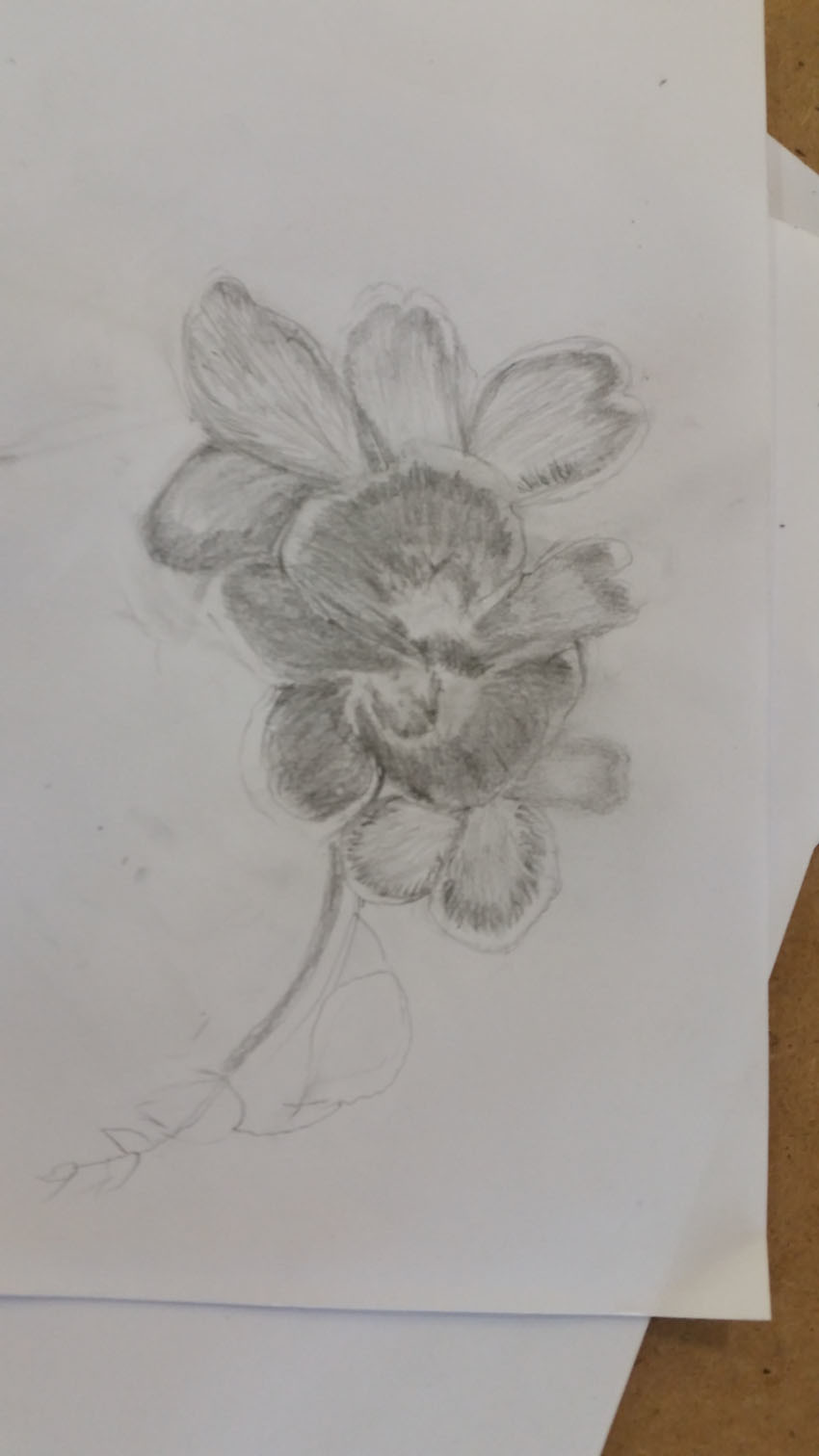A meticulously detailed pencil drawing of a flower is positioned on a white piece of paper. The sketch features intricate shading and outlines, capturing a flower with numerous petals and leaves. While the exact species of the flower is unclear, the artist's use of pencil creates a compelling blend of gray tones that bring the image to life. This primary sheet rests on top of two other pieces of paper, haphazardly stacked beneath it, contributing a sense of casualness to the scene. These papers are laid on a surface with visible brown hues, suggesting a wooden table beneath. The brown tones peek through predominantly on the right-hand corners at both the top and bottom of the arrangement, providing a subtle but warm contrast to the grayscale drawing.